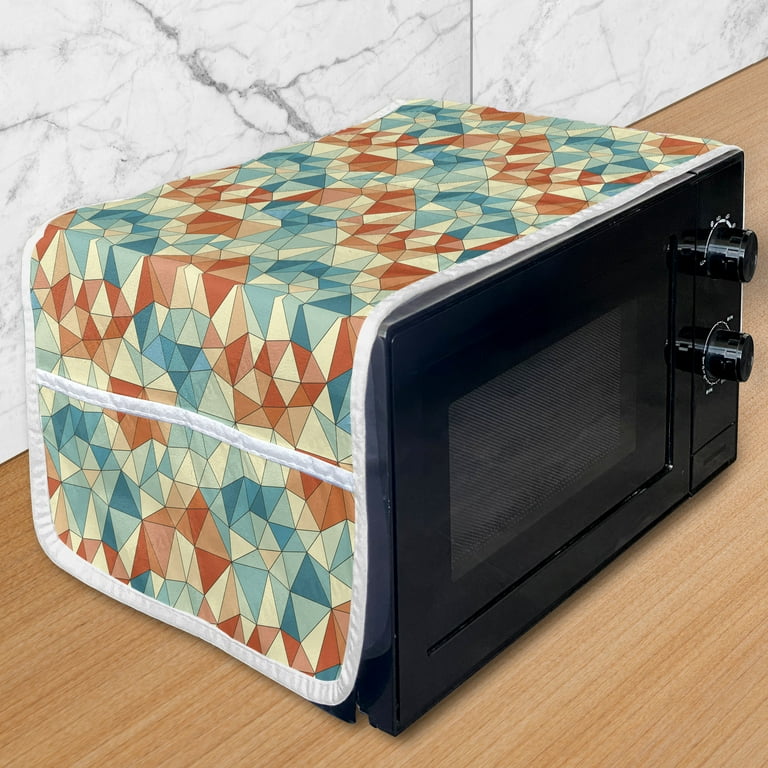This photograph captures a black microwave situated on a wooden countertop, with a granite backsplash featuring white marble-like patterns and black veins in the background. The microwave, which has a small window on its front, is equipped with two knobs—the top one likely for controlling the time and the bottom one potentially for adjusting the power level. Draped over the top and partially down the sides of the microwave is a colorful fabric cover featuring a vibrant tessellation of red, blue, yellow, light blue, and orange geometric shapes such as triangles, diamonds, and trapezoids. This cover also includes a small pocket, suggesting functionality for storage. Notably, the cloth does not obscure the front face, leaving the window and dials visible.